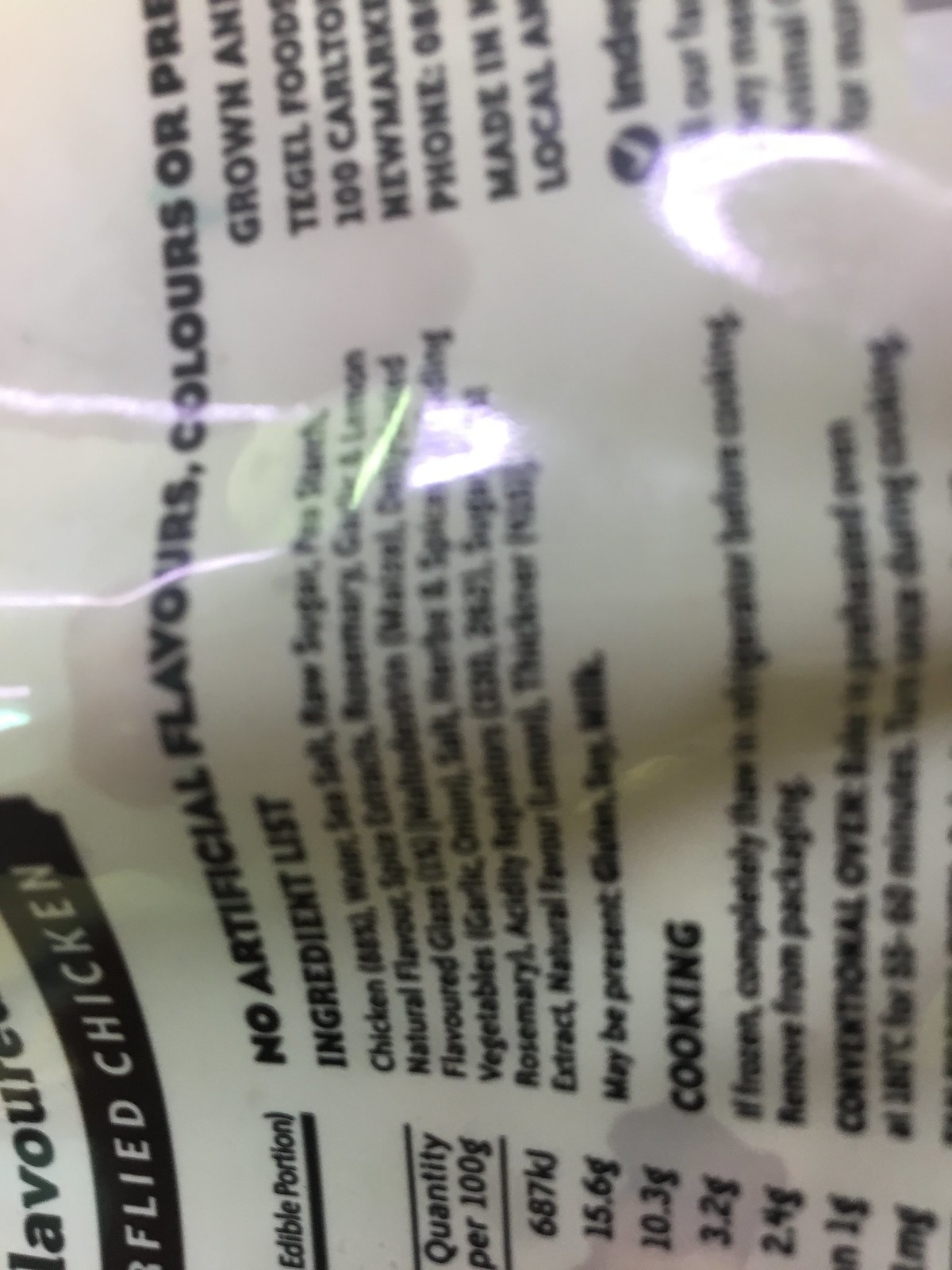A close-up view of the back of a white plastic package, zoomed in to show the text detailing nutritional information and cooking instructions. The black text is slightly blurred but indicates no artificial flavors or colors. The visible portion lists ingredients starting with 'chicken' and other partially obscured items. The package is oriented sideways in the image, with the top facing the left.